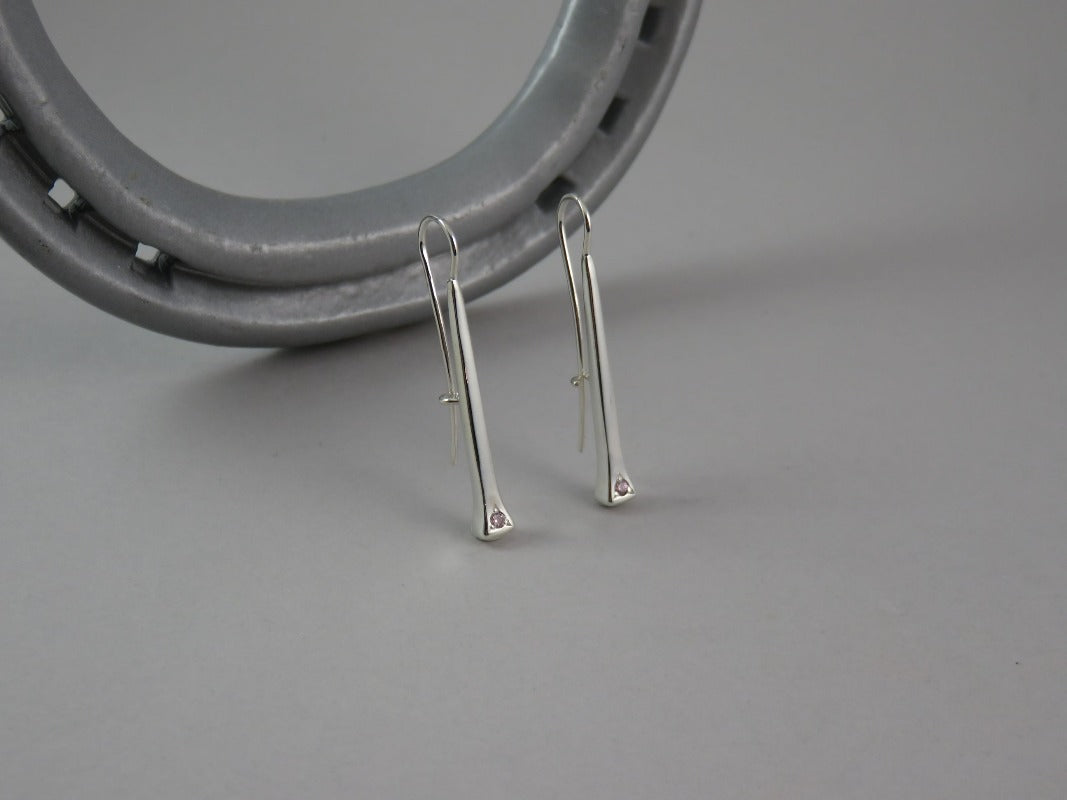This is a detailed color photograph in landscape orientation, prominently featuring a pair of horseshoe nail drop earrings against a medium gray background. The earrings are positioned in the center of the image, leaning against a dark gray metal horseshoe that enters the frame from the top left and is partially cut off. The horseshoe, with its curved U-shape and holes reminiscent of a traditional horseshoe, is bolted to the surface, adding a rugged texture to the composition. The earrings themselves are silver, with a reflective sheen and a flared nail design at the bottom. They are adorned with small, light pink jewel-like dots at their bases and are equipped with silver French loops at the tops, creating a delicate yet industrial aesthetic. This photograph embodies the style of photographic representationalism, realism, and product photography, capturing the fine details and textures of both the earrings and the horseshoe backdrop.